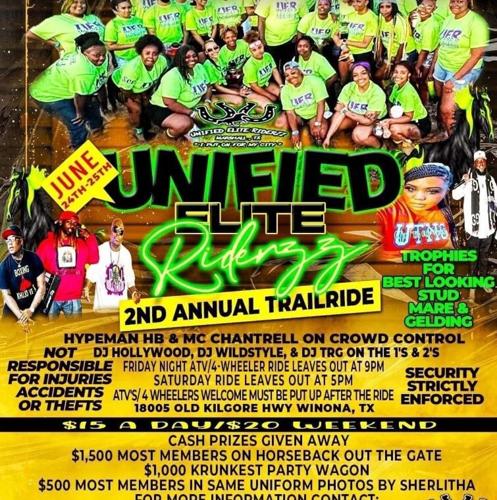This is an image of a colorful flyer advertising the "Unified Elite Riders 3," for their second annual trail ride event, taking place on June 24th and 25th. The event title, "Unified Elite Riders 3," appears prominently with "Riders 3" in neon green text and "Unified Elite" in black text outlined in green at the top of the flyer. 

At the top of the flyer, a photo features a group of women wearing neon green shirts, posing together, presumably members of the Unified Elite Riders. The middle section of the flyer provides several key details about the event, such as the cost ($15 per day or $20 for the whole weekend) and the offering of cash prizes. 

It also mentions that trophies will be awarded for the best-looking stud, mare, and gelding, indicating a focus on horse riding activities. Moreover, there is important information about regulations: all ATVs and four-wheelers must be put up after the ride, and the event organizers are not responsible for any injuries, accidents, or theft. Security measures will be strictly enforced, and there are pictures of the DJs who will be performing at the event. The flyer has a homemade appearance and might typically be found on a telephone pole or similar public place.